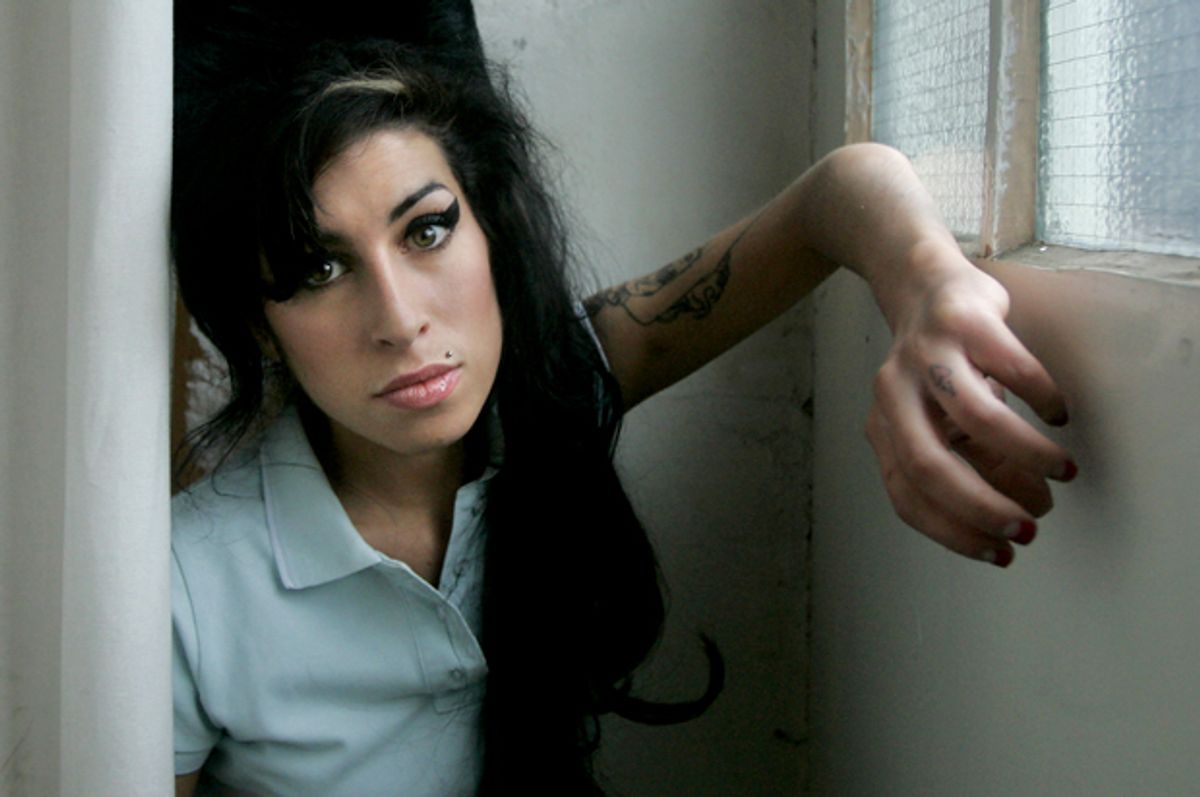In this evocative photograph of Amy Winehouse, she is seen beside a window within a dilapidated, white-tiled bathroom, featuring aged, cracked walls with darker stains accentuating the wear. On her left, a plastic shower curtain partially obscures the room. Amy is positioned with her back against an opaque, wire-reinforced window that hints at the stark, institutional feel typical of a hospital or mental health facility. She wears a very light sky blue, collared polo shirt, open at the neck, showcasing her iconic beehive of thick black hair and heavily applied winged eyeliner, along with her distinctive mole above her pink lips and lip piercing. Her left arm is raised and bent against the window, revealing a glimpse of her tattoos on her arm and ring finger, while she gazes solemnly yet intently at the camera, her expression capturing the raw essence of her famed soulful persona.